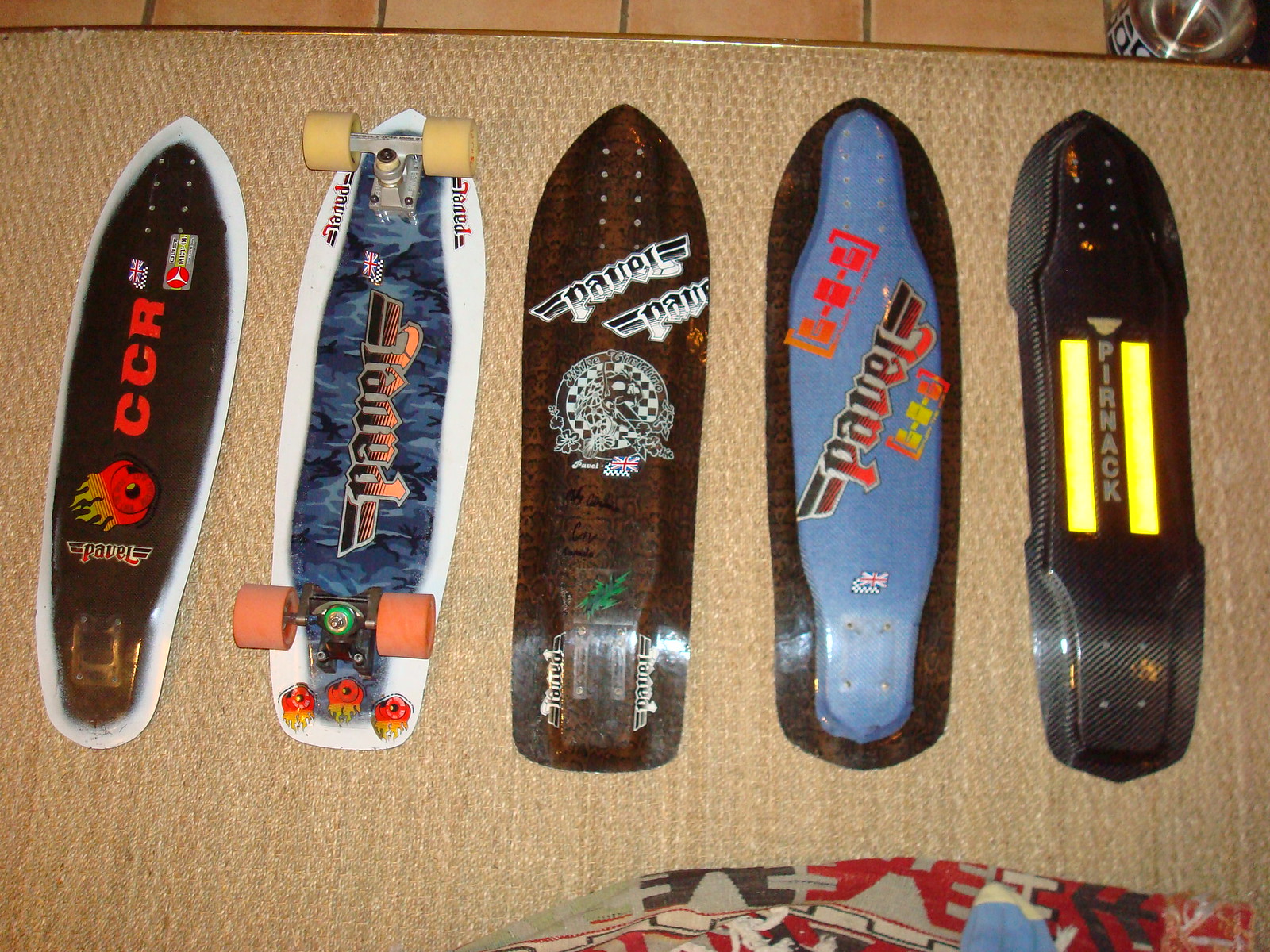The image showcases five skateboards laid out upside down on a brown, diamond-patterned carpet, which transitions to a brown tile-like floor. All five skateboards are positioned side-by-side, with one skateboard featuring wheels while the others are without. From left to right, the first skateboard is black with a fiery wheel graphic and red lettering that reads "CCR." The second skateboard is brown with black lettering spelling "PAVEL." Next in line, the third skateboard also reads "PAVEL" in red font on a blue background with black edging. The fourth skateboard is primarily black with bold yellow rectangles and the lettering "PIRNACK." Finally, the fifth skateboard shows a white deck with tan and light orange wheels and some indistinguishable lettering.